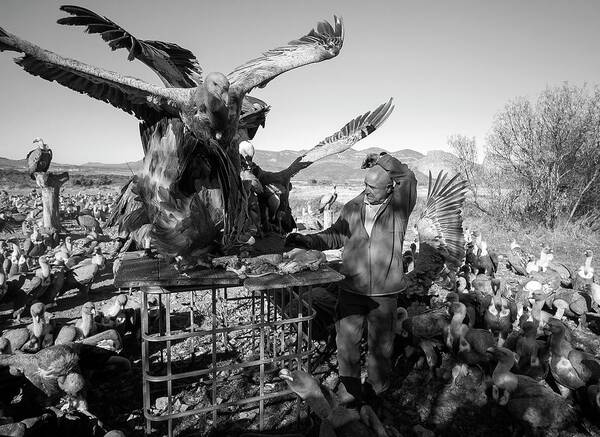The black-and-white photograph depicts a balding man wearing a jacket over a polo shirt, with jeans and boots, standing in an open, flat area with a bush in the near distance and mountain tops visible far off. The man, with his right arm resting over his bald head, appears to be feeding or attending to a large number of vultures. In front of him, three large vultures, wings spread, stand on a table supported by a metal stand, while dozens of baby vultures surround his feet, vying for his attention and the meat he is placing on the table. Additional birds, including pigeons, turkeys, and even what appears to be a peacock, densely populate the area, creating an intriguing scene of chaotic avian activity.